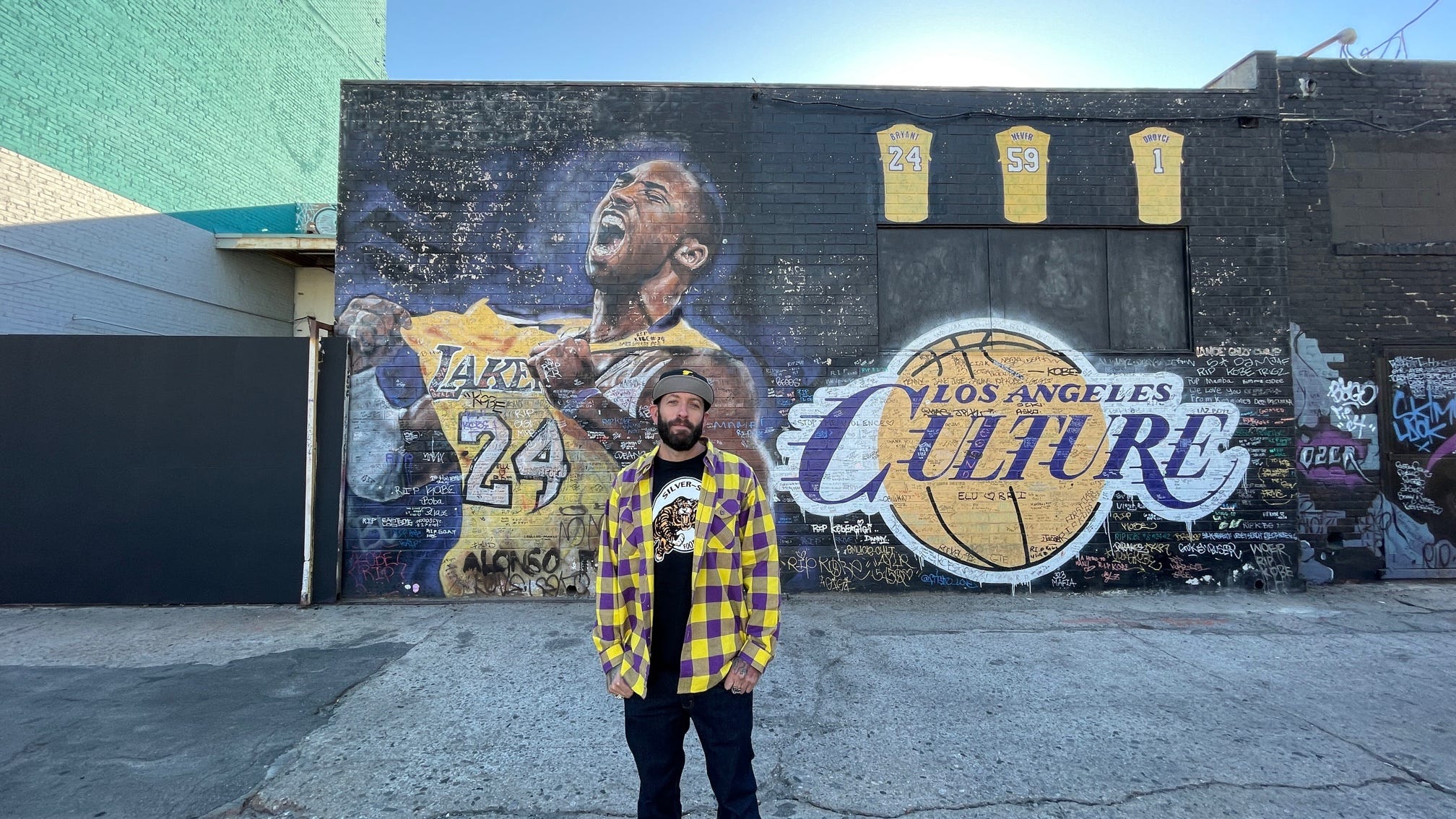In this vibrant outdoor photograph taken in bright natural lighting, a mural of Kobe Bryant commands the scene, painted on the side of an old, black brick building. The sky above is clear and blue, adding a serene backdrop to the intense portrait. Kobe Bryant is depicted mid-roar, his head tilted back, eyes squeezed shut, and mouth wide open in a triumphant scream. He is clad in his iconic yellow Lakers jersey, number 24, gripping and pulling it away from his chest. A white sleeve adorns his right arm. To Kobe's right, the mural features a large yellow basketball with bold purple text reading "Los Angeles Culture," situated just above a boarded-up window. Above this, three painted jerseys, numbered 24, 59, and 1, hover as a tribute. 

In the foreground, directly in front of the mural, stands a man with a commanding presence. He sports a black baseball cap accented with yellow lettering, a thick black beard, and wears a checkered purple and gold flannel shirt which is unbuttoned to reveal a black and white t-shirt underneath. His ensemble is completed by black pants. The cracked and worn concrete ground beneath him reinforces the aged ambiance of the setting.